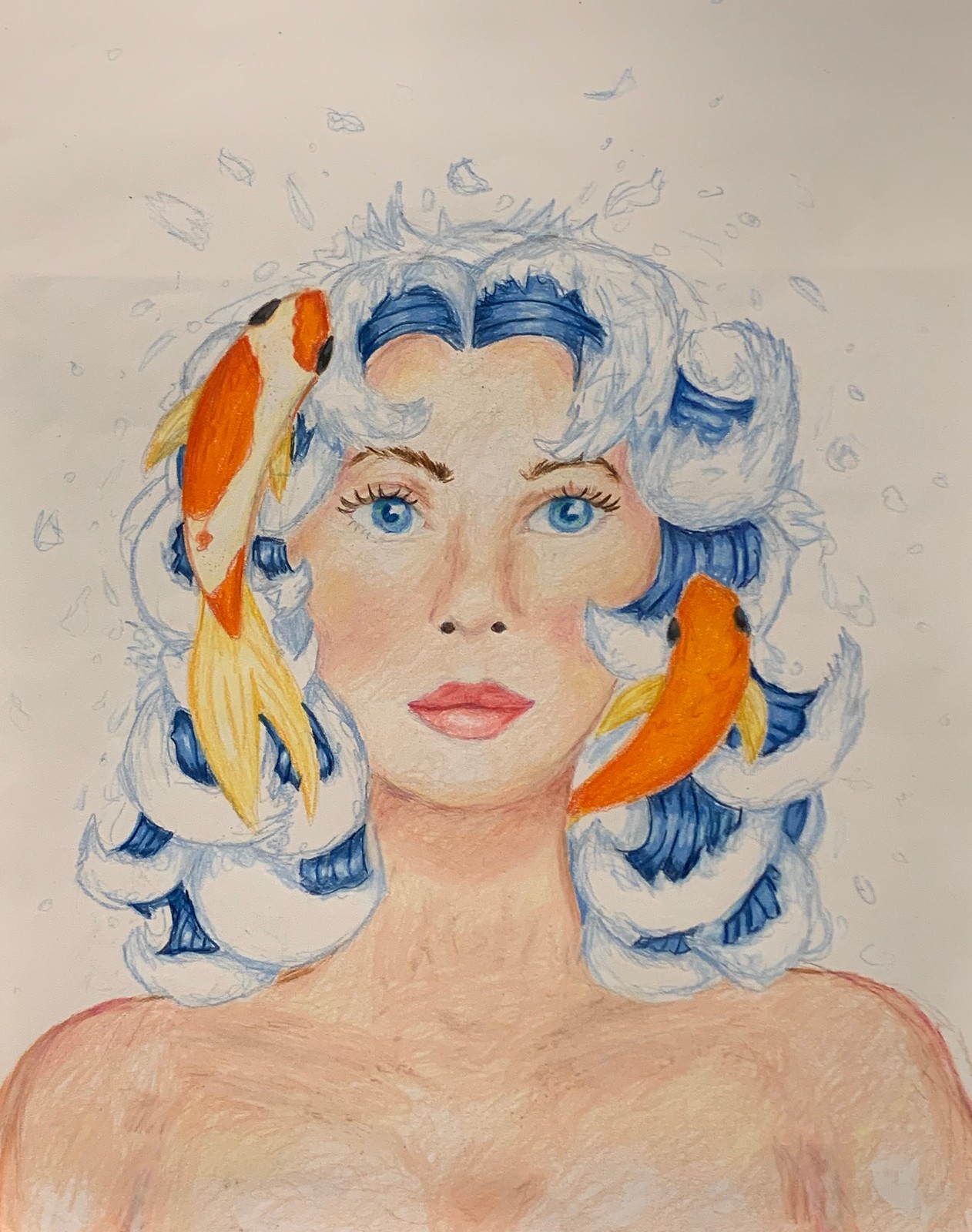The image is a detailed artwork of a woman in portrait style, focusing on her head and shoulders against a white background. She has striking blue eyes with dark blue pupils, and her eyebrows are brown. Her white hair flows like sea waves, accentuated by splashes of water, emphasizing an aquatic theme. Integrated into her hair are two goldfish, one on each side; the fish on the right has yellow fins, while the one on the left features a mix of orange and white with yellow fins. The woman has light skin and red lips, and she appears to be topless, with portions of her chest visible at the bottom of the image. No additional text or figures are present in the artwork, and the woman gazes directly at the viewer, enhancing the intimate and unique oceanic essence of the piece.